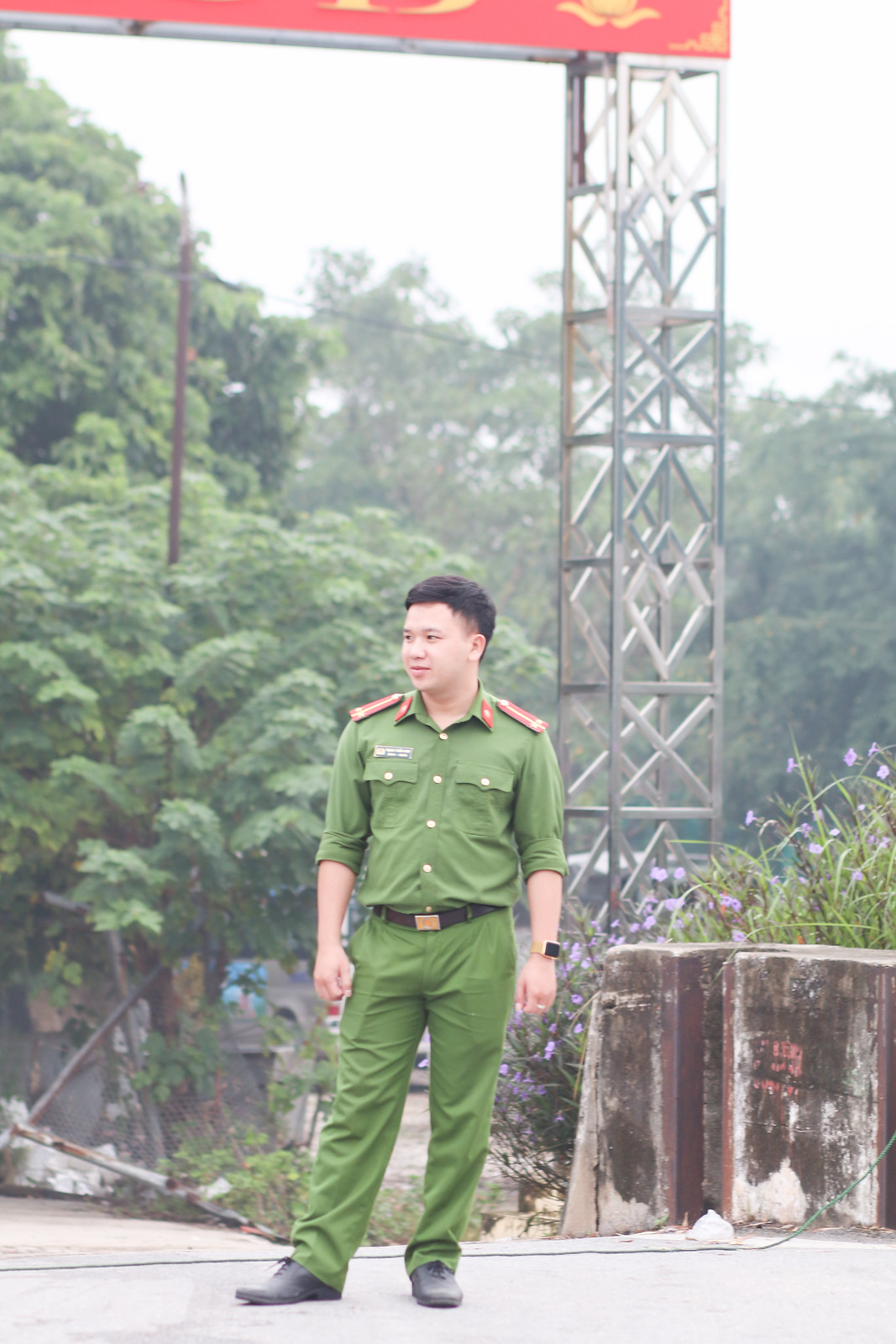In this outdoor daytime photographic image, a young Asian man is prominently featured, wearing a green military uniform adorned with red and white epaulets. His uniform includes notable red and yellow collar markings and an unreadable name tag over his left breast. He also sports a black wristwatch with a black face and the outline of a smartphone is visible in his pants. His attire includes a black pair of pants and a black belt with a gold buckle. The man, with very short hair, is looking slightly to his left.

He stands on a sidewalk next to a metal tower, possibly telephone scaffolding. To his right, there are a couple of gray pillars with unreadable Asian writing. The background reveals a dull gray sky, lots of trees, and a hint of a blue vehicle or object amidst the cluttered scene.